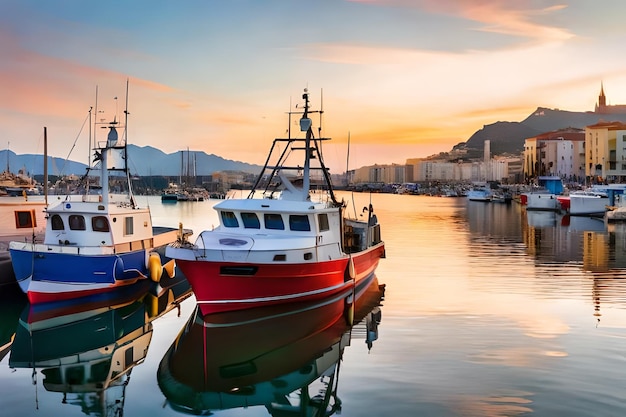This photograph captures a serene harbor scene reminiscent of the Mediterranean with a calm, still body of water reflecting the surrounding beauty. In the background, charming buildings with Mediterranean architecture are framed by distant mountains, evoking a picturesque landscape. The sky, painted with the soft hues of an impending sunset, adds a warm, tranquil ambiance to the scene.

In the foreground, a distinctively shaped boat with a pointed red bottom and a white cabin dotted with numerous windows takes center stage. This vessel, sharp and almost toy-like, features towers atop its structure. Adjacent to it on the left, a similar boat boasts a mostly blue bottom, accentuated with a white stripe and a red band beneath it. Both of these boats are prominently positioned, offering a clear, striking reflection on the water's undisturbed, dark surface. The water itself is so still that it mirrors the sky’s orange and yellowish tones, creating a harmonious blend of sky and sea. Additional boats can be seen further back, adding depth and context to the peaceful harbor scene.